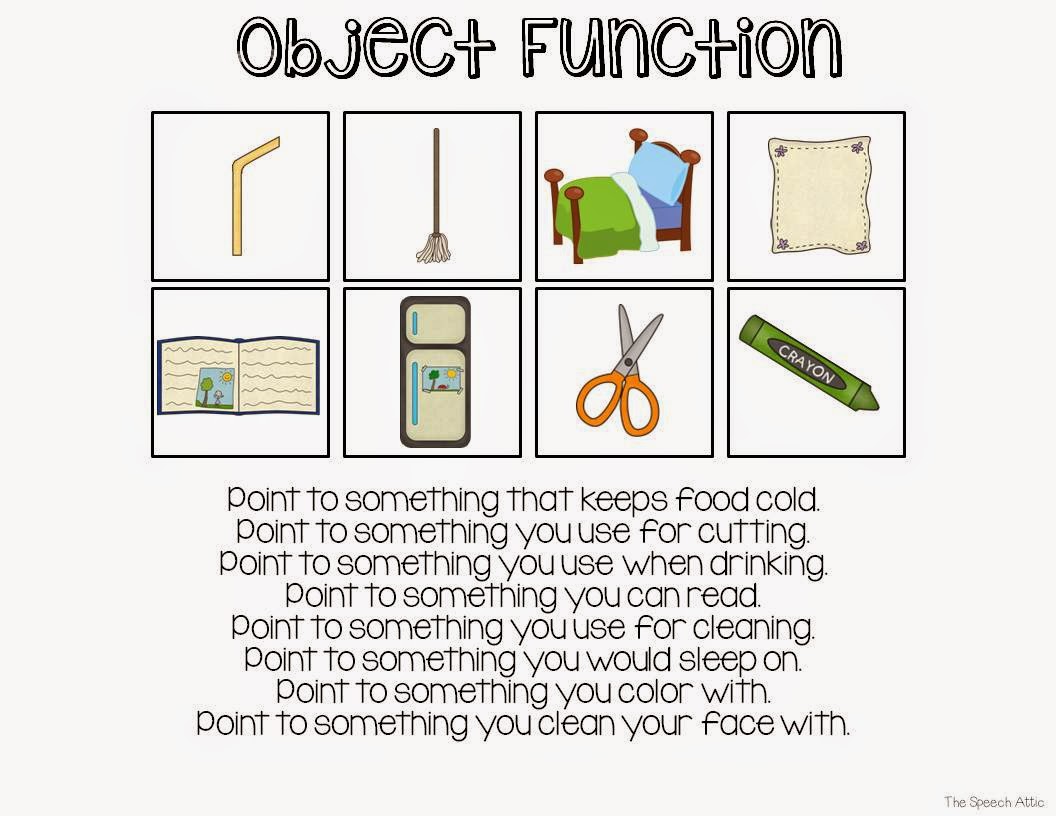The image is a rectangular educational aid for children, slightly wider than it is tall, measuring approximately six inches in width and five inches in height. The background is a pale gray, almost white. Positioned at the top center, the bold text "Object Function" is displayed with a black outline, prominently featuring uppercase letters for "O" and "F".

Below the title, there are two rows of squares, each containing four cartoon-style objects against light-colored gray backgrounds, organized in a grid. The top row includes a yellow straw, a broom, a bed, and what appears to be a handkerchief or pillowcase. The second row features an open book, a refrigerator, a pair of scissors, and a green crayon.

Underneath these objects, black-print instructions prompt the viewer to identify items based on their functions: "Point to something that keeps food cold. Point to something you use for cutting. Point to something you use for drinking. Point to something you can read. Point to something you use for cleaning. Point to something you would sleep on. Point to something you color with. Point to something you clean your face with."

This comprehensive description highlights shared details and emphasizes the educational nature of the image, which aims to help children learn about the uses of everyday items.